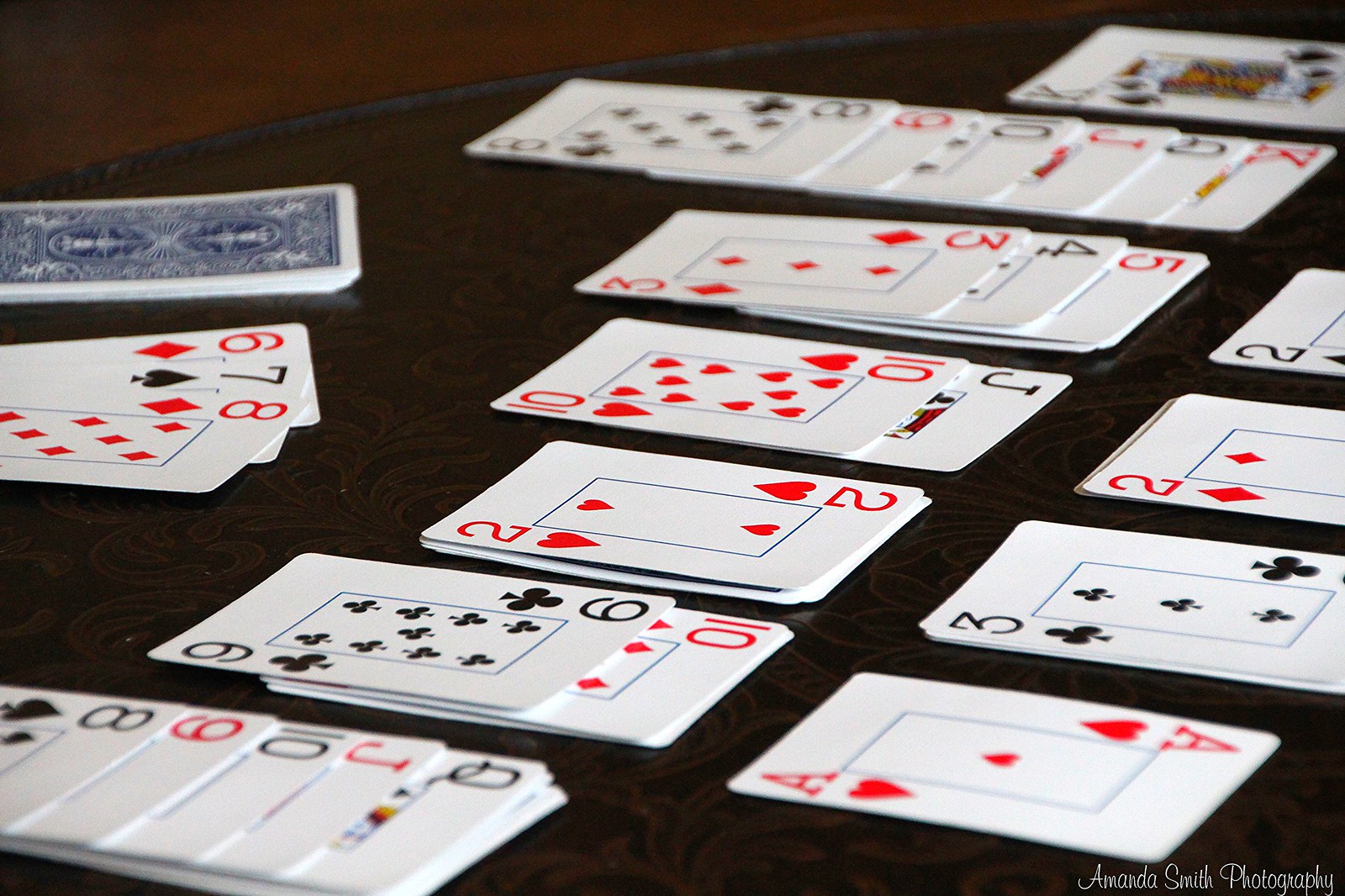The photograph captures an intricate layout of solitaire, also known as patience, being played on a dark black table. The cards are arranged in a visually striking diagonal pattern from the top right-hand corner to the bottom left-hand corner. 

- The topmost row features a solitary King card. 
- The second row down showcases a King, Queen, Jack, and the sequence 10, 9, and 8.
- The third row holds the numbers 5, 4, and 3.
- The fourth row consists of a Jack and a 10.
- The fifth row is represented by a single card numbered 2.
- The sixth row presents both a 10 and a 9.
- The bottom left-hand edge displays a sequence of Queen, Jack, 10, 9, and 8 cards.

In the foreground, three cards (6, 7, and 8) are fanned out impressively, positioned just in front of a stack of upside-down cards. Additionally, running vertically down the right-hand side of the image are cards numbered 2, 2, 3, and an Ace.

The elegant signature "Amanda Smith Photography" is inscribed at the bottom right-hand corner, completing the image with a professional touch.